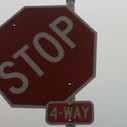This is a small, slightly blurry photograph taken on a cloudy day, featuring a standard red, octagon-shaped stop sign with white lettering that reads "STOP." The stop sign is attached to a metal pole and appears to be leaning to the left because the top screw is missing. Below the stop sign, there is a properly aligned, smaller rectangular sign that reads "FOUR-WAY" in white letters on a red background, indicating a four-way stop. The background of the image is a light gray, likely due to the overcast sky, and the overall lighting of the photo is dim.